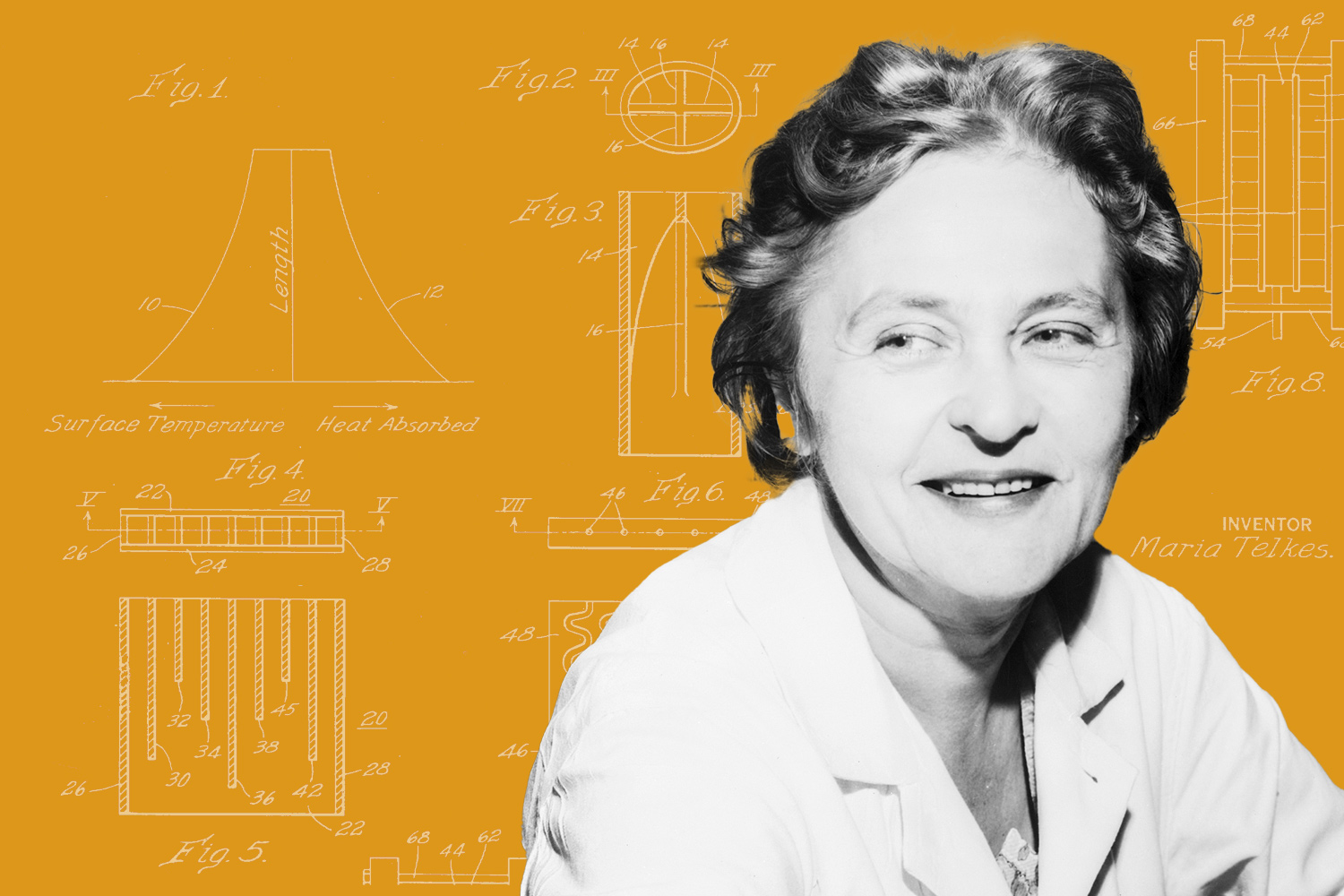This is a detailed black-and-white photograph of middle-aged inventor Maria Telkes, wearing a white lab coat and smiling as she looks off to her right. She has short, wavy hair that falls just below her ears, well-defined eyebrows, and a warm smile that reveals her teeth. The background merges an orange hue with white technical drawings, showcasing eight numbered figures, labeled from one to eight. These diagrams, which appear to be engineering designs, include handwritten notes, measurements, and charts, reflecting various inventions and projects from her career. The orange backdrop with white sketches stands out, presenting a visually engaging contrast to her monochromatic portrait. Her name, Maria Telkes, is also visible in the background, affirming her identity as the notable inventor.